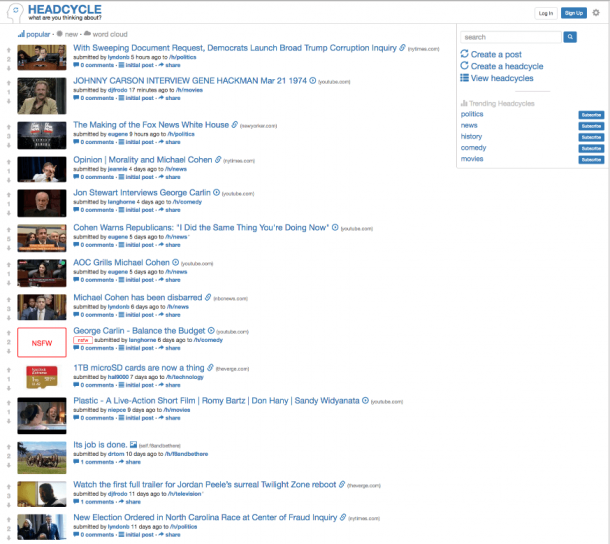The image features a digital interface titled "Head Cycle" prominently displayed in blue text at the top left, denoting a website or application. Central to the image is a stylized graphic of a head, facing left, encircled by blue arrows suggesting a cycle of thoughts or ideas. Below the head cycle graphic, the tagline reads, "What are you thinking about?"

The interface is divided into several topical categories: Popular, New, and White Cloud. In this image, "Popular" is highlighted in blue, indicating it is the selected category.

The following headlines are listed under "Popular":

1. **Which sweeping document request Democrats launched brought Trump corruption inquiry?**
2. **Johnny Cassin interview with Jane Heckman, March 21, 1974.**
3. **The Making of the Fox News White House.**
4. **Opinion: Morality and Michael Cohen.**
5. **Jon Stewart interviews George Killeen.**
6. **Cohen wants repayments: "I did the same thing you are doing now."**
7. **AOC Grills Michael Cohen.**
8. **Michael Cohen has been disbarred.**
9. **George Killeen Balanced the Budget.**
10. **One Terabyte Micro SD Cards Are Now a Thing.**
11. **Plastic, a Life Exchange: "What feeling wrongs, but it doesn't hurt."**
12. **Sandy, We Do Not.**
13. **This Job is Done.**
14. **Watch the First Full Trailer of Jordan's Palace - Shuttle Toilet Zone Reboot.**
15. **New Election Ordered in North Carolina Race Amidst Fraud Inquiry.**

All headlines are presented in blue text, maintaining uniformity in design. At the top right of the interface, options including "Create a Post," "Create a Head Cycle," and various categories like Politics, History, Comedy, Movies, and Trending are visible. A "Sign Up" button is also prominently displayed in the top right corner, inviting user engagement.